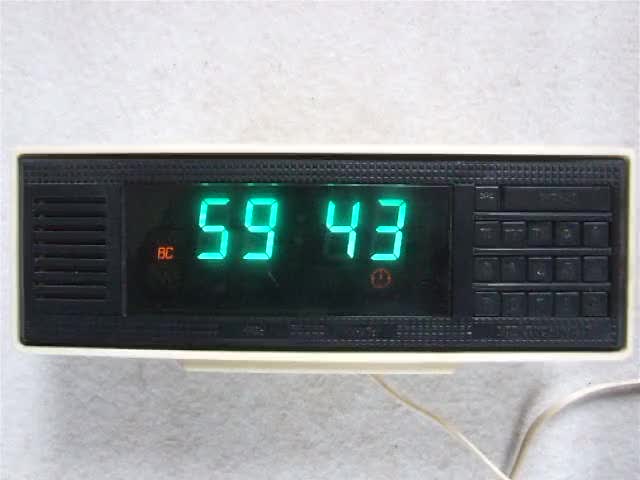The image depicts an old-school digital clock with a rectangular shape, featuring a black face and cream-colored trim. Central to the clock is a glowing digital readout displaying "59:43" in a cool aqua color, potentially indicating a timer set for 59 minutes and 43 seconds. Beneath these digits, there is a small clock symbol, suggesting its dual function. To the left of the digits, in small reddish-orange letters, is the label "BC". The clock is adorned with approximately 20 various buttons, primarily square-shaped with one prominent rectangle at the top. Positioned on the far left side is a speaker with slotted openings. The clock includes a white cord trailing from its base, indicating AC power supply. All of this is set against a white shelf, with a neutral gray, possibly stucco, background.